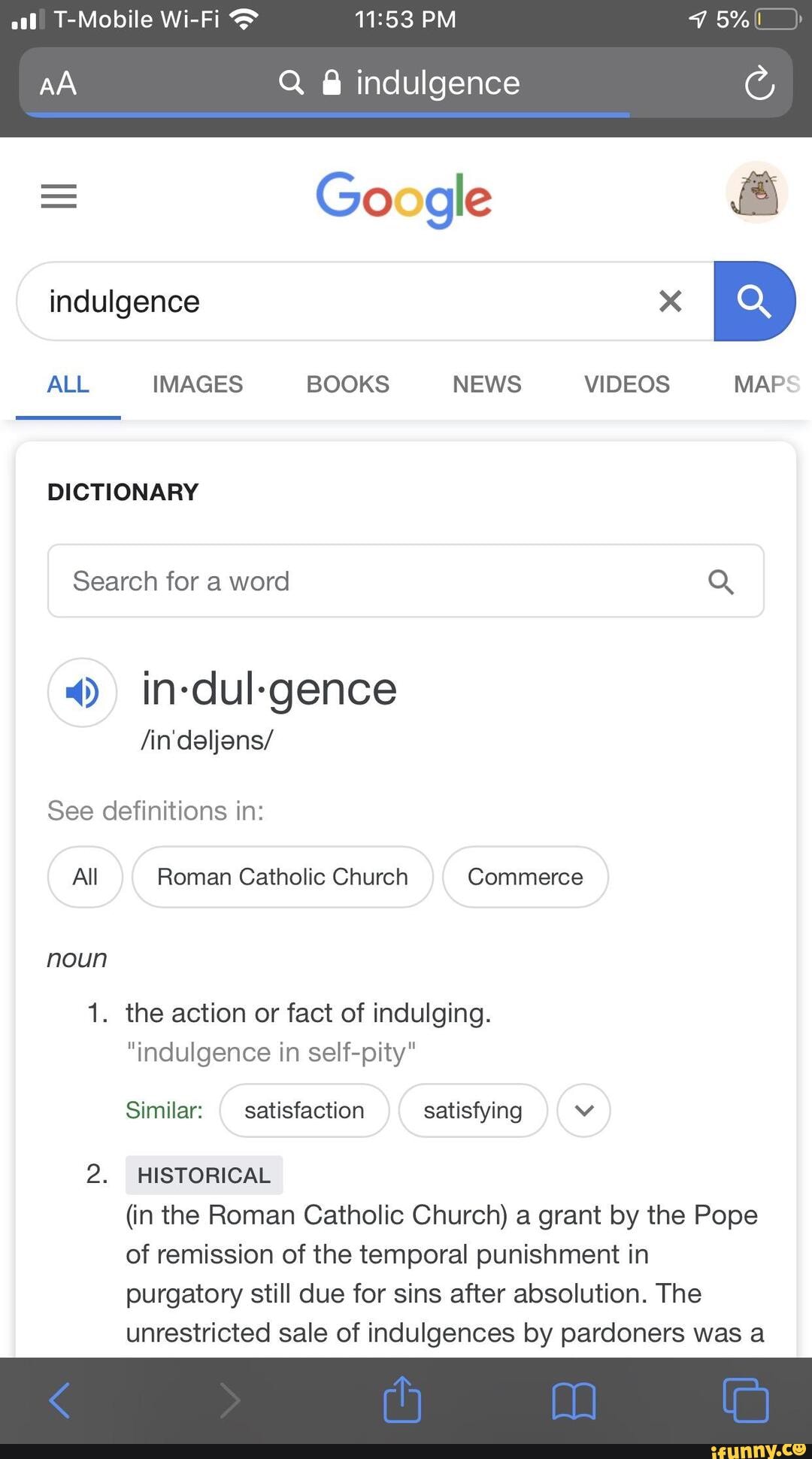In the image, we see a screenshot taken from a mobile device, either a tablet or a phone, distinguished by the presence of status icons along the top border. These icons include indicators for T-Mobile service, a Wi-Fi connection, the time reading 11:53 p.m., and a critically low battery level at 5%.

Center stage in the screenshot is a Google search results page, indicating the term "indulgence" has been entered into the search query. The interface displays typical Google search elements: an "X" mark to clear the entry, a magnifying glass icon for the search function, and various tab options such as 'All,' 'Images,' 'Books,' 'News,' 'Videos,' and 'Maps.'

Directly under the search field, the search results commence with the dictionary definition of the word "indulgence." This section clarifies the term through multiple lenses: a general definition, a Roman Catholic Church-specific definition, and a commerce-related context. The primary definition offered is: "the action or fact of indulging," exemplified in the phrase "indulgence in self-pity." Synonyms listed include "satisfaction" and "satisfying."

Further down is a historical note, which explains the term in the context of the Roman Catholic Church as a "grant by the Pope of remission of the temporal punishment in purgatory still due for sins after absolution." However, the text cuts off and is not fully visible, ending with a partial sentence: "the unrestricted sale of indulgences by part of the nurse was a..."

The screenshot's focal point revolves around providing a comprehensive view of the search results for "indulgence," primarily dominated by the word's dictionary definitions.